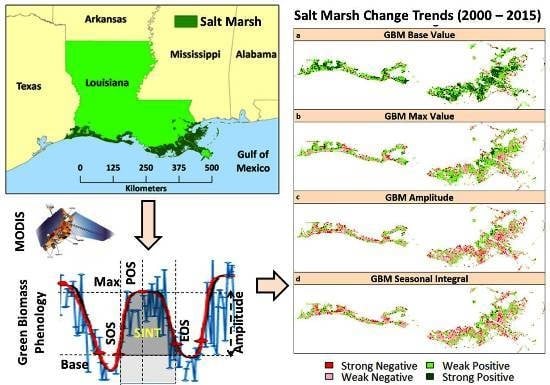This image is a detailed and color-coded scientific diagram divided into three sections, focusing on salt marsh changes and their trends between 2000 and 2015, specifically in Louisiana. 

On the top left, there is a blue and pale yellow map highlighting several southern U.S. states—Texas, Arkansas, Louisiana, Mississippi, and Alabama—with Louisiana prominently filled in bright green. This map indicates salt marsh areas along the Louisiana coast, labeled "salt marsh." Below the map is a graph titled "Green Biomass Phenology," represented in blue and grey with vertical text on the side. This section includes a line graph measuring changes over time.

On the right-hand side, under the heading "Salt Marsh Change Trends 2000-2015," there are four graphs outlined in green and orange, showing various salt marsh trend measurements over the years. The graphs measure GBM (Green Biomass) base value, max value, amplitude, and seasonal integral. Each graph has a pale orange background heading. Below these graphs, a legend explains the color codes used: red signifies "strong negative," beige indicates "weak negative," green represents "weak positive," and black stands for "strong positive."

The diagram is interconnected by arrows: one from the top-left map to the bottom graph, and another from this graph to the section on the right. The visual representation of data helps illustrate the changes in Louisiana's salt marshes over the specified period.